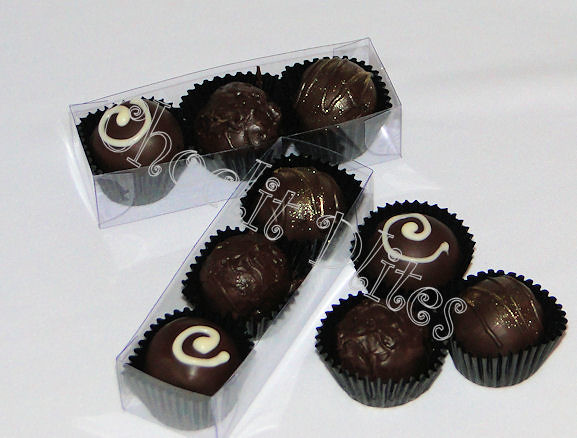Displayed in front of me is a vibrant color photograph featuring delectable chocolate truffles styled as an advertisement for a product called Chocolate Delights, notably spelled 'C-H-O-C-L-I-T, D-L-I-T-E-S.' The truffles rest atop a pristine white tablecloth, their rich, glossy appearance highlighted by the precise lighting. 

Each truffle is presented in elegant black paper cups that resemble mini cupcake holders, adding a touch of sophistication. There are two clear plastic packages, each containing three truffles, perfectly arranged for sale. Three additional truffles are displayed outside the packages, two are solid chocolate while one boasts an enticing white vanilla swirl on top. 

The chocolates exude a dark, luxurious sheen with decorative swirls and a light dusting of sparkling sugar. Cutting through the center of the photograph in white-outlined font is the word "Chocolates," drawing focus to the treats below. The letter "C" also subtly mirrors the swirl design found on some of the truffles, enhancing the cohesive branding throughout the image. 

In total, there are nine truffles depicted, grouped neatly into threes, either within their clear packaging or showcased individually on the table. This enticing display captures the allure of these chocolate desserts, making them appear irresistibly tempting.